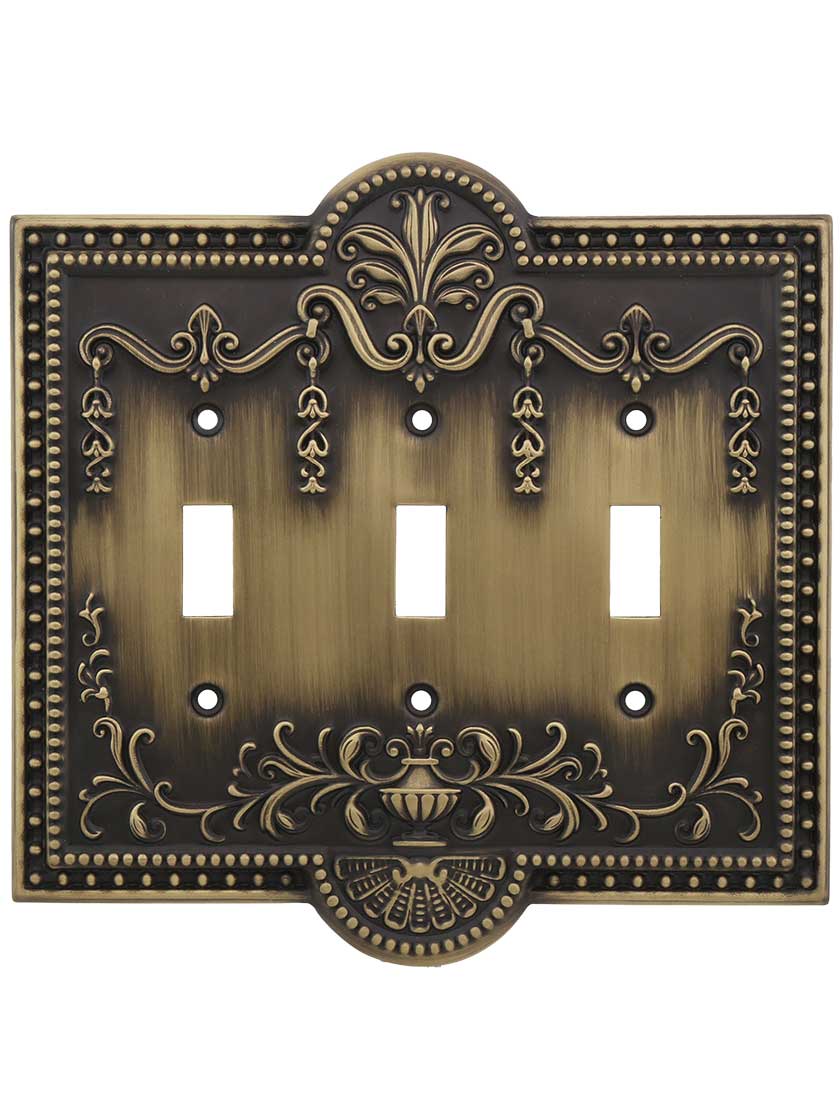This color photograph showcases an intricately designed light switch plate cover, fashioned from a brass-like metal with a brushed texture. The oblong, square frame is adorned with an ornate floral and leaf pattern, featuring detailed carvings reminiscent of bronze and black hues. It has a distinct rounded crest at both the top and bottom middle sections, and a series of small dots bordering the entire piece. The plate is designed to accommodate three light switches, with rectangular openings evenly spaced in the center and round holes above and below each opening for screws. At the top, a tree motif is prominently carved, enhancing the decorative appeal. The photo contains no writing, people, animals, or additional structures, focusing solely on the switch plate's detailed craftsmanship.